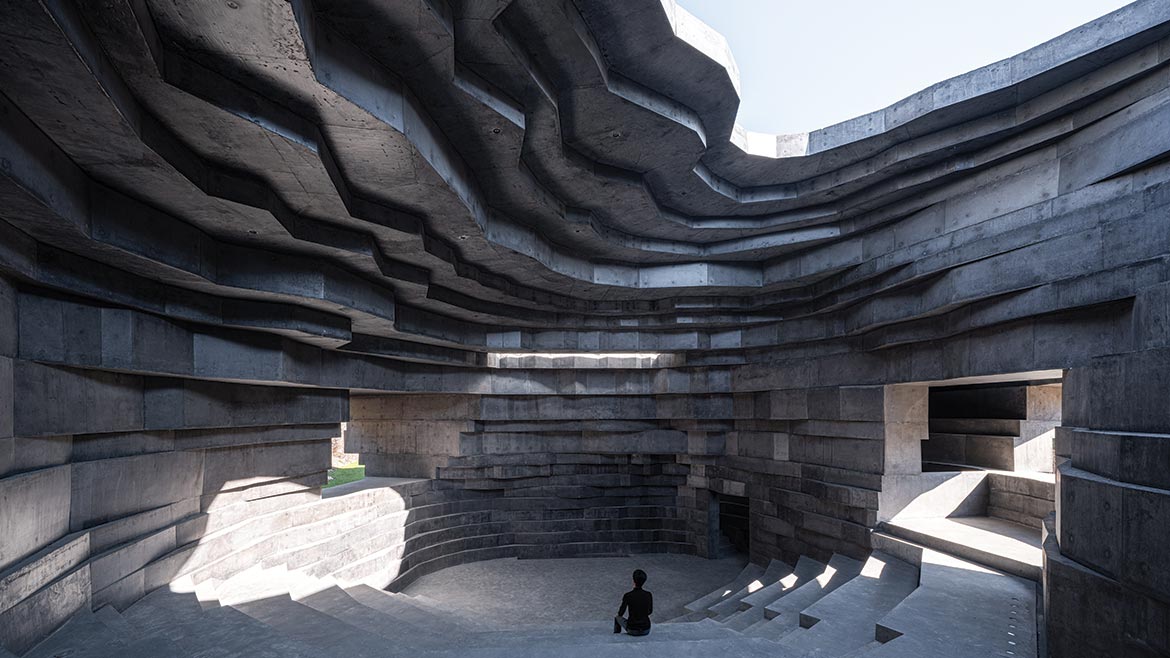The image depicts a computer-rendered interior space resembling a meticulously designed artificial canyon or cavern. This horizontally oriented scene showcases a small auditorium crafted from layers of smooth rock or cement blocks, creating a tiered seating arrangement around a central core that serves as the stage. The open ceiling and entryway allow natural light to illuminate the space, adding to its serene and contemplative atmosphere. A solitary human figure, silhouetted in black, sits on one of the raised seating areas, gazing into the empty cavern. The structure has a modern, geometric aesthetic, with straight lines and smooth surfaces that suggest it is an artificial construct, possibly created with a VR or graphics program. To the right, an opening leads to adjacent rooms featuring similar layered seating. This quiet, meditative environment combines elements of an auditorium and a sanctuary, evoking a sense of tranquility and introspection.